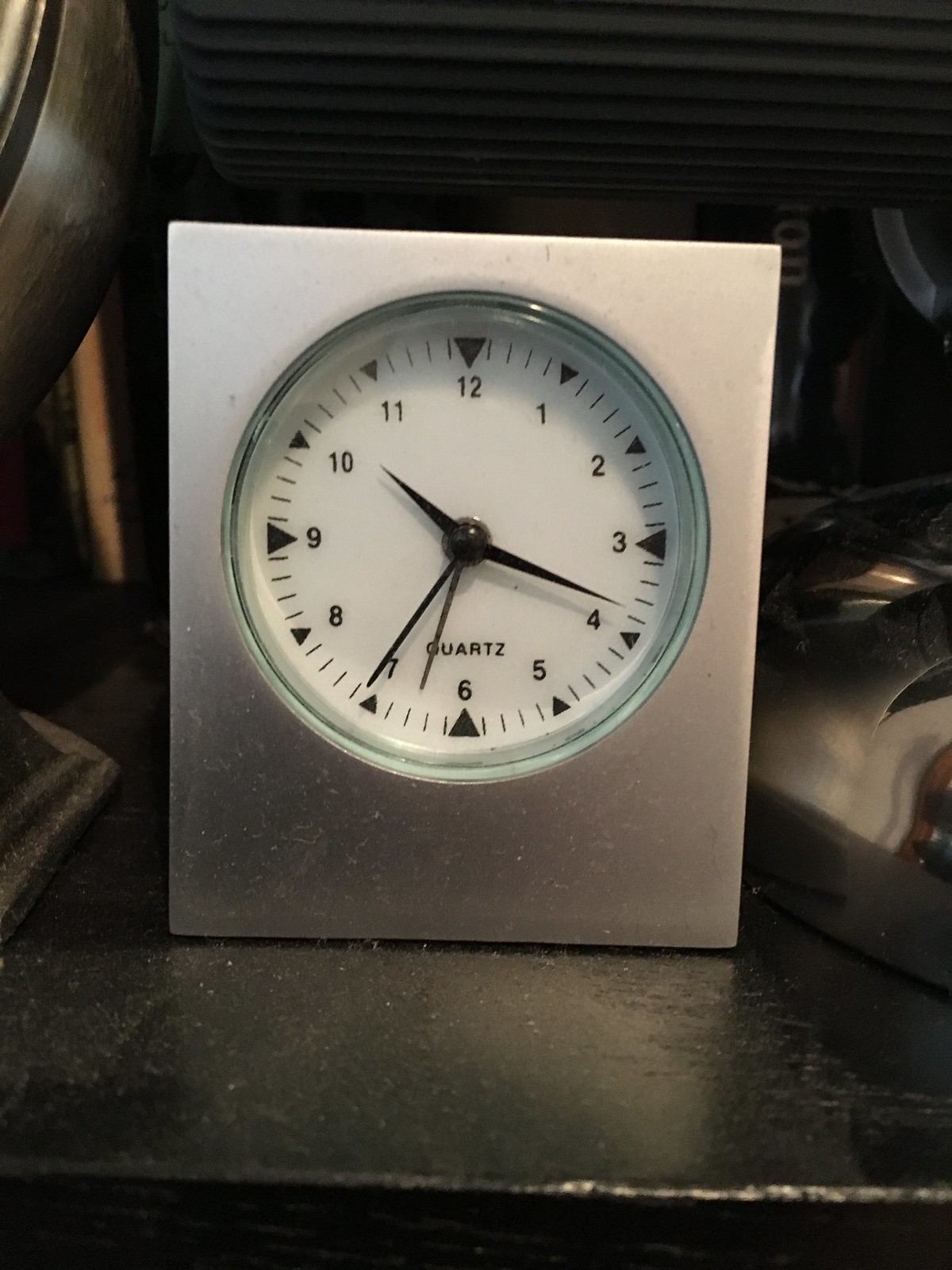This photograph features a meticulously designed wall clock, set within a gleaming silver frame reminiscent of a picture frame. The face of the clock is protected by a clear plastic cover, revealing a pristine white background. Bold black numerals are displayed prominently from 12 through 11, each accompanied by a corresponding triangular marker. Between these numerals, small black dashes mark the individual minutes. The clock is equipped with three sleek black hands – hour, minute, and second – creating a sharp contrast against the white backdrop. Notably, the word "QUARTZ" is emblazoned in uppercase letters near the 6 o'clock position, underscoring the clock's precise timekeeping mechanism. The overall design is a striking interplay of monochromatic tones, blending simplicity and elegance.